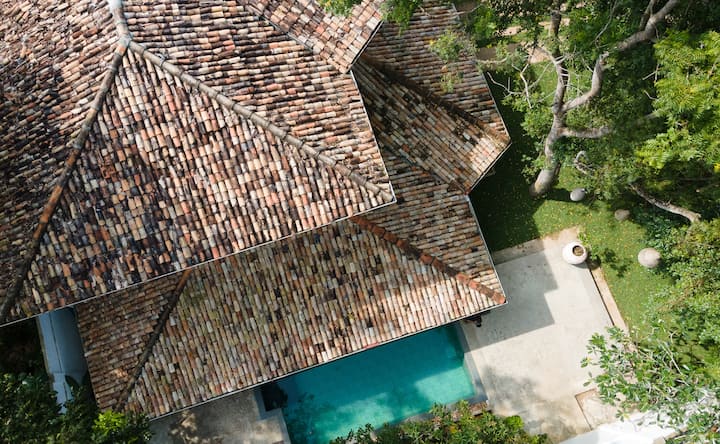This aerial photograph, likely taken by a drone, showcases a unique view of a house and its backyard with detailed elements. Dominating the upper left portion of the image is a distinctive tricolored tile roof. The tiles, resembling little round beads, are a mix of beige, brown, and dark brown, evoking an arrangement akin to kernels of corn. The roof, which is highlighted at the peaks and shadows, appears to extend and form a point at the top, possibly influenced by either American or Japanese architectural styles.

To the right of the house, a tall tree with light gray, slightly curved branches and lush green foliage captures the eye. Beneath the tiled roof, centrally in the image, lies a rectangular pool with a light blue, aquamarine bottom. This pool is bordered by a clean, white concrete patio that forms a slightly notched, rectangular shape. On the right corner of the patio, there's a round, ceramic vase filled with green foliage, blending harmoniously with the small surrounding lawn.

The lawn, dotted with a few small smooth rocks, lines the garden with additional green grass, adding a natural touch to the structured elements. Close to this garden space, there is a tan-colored dirt path in the background and a white board or fence along the left side, providing a framed boundary. The composition of roofs, foliage, and structured elements creates an intricate and inviting backyard scene.